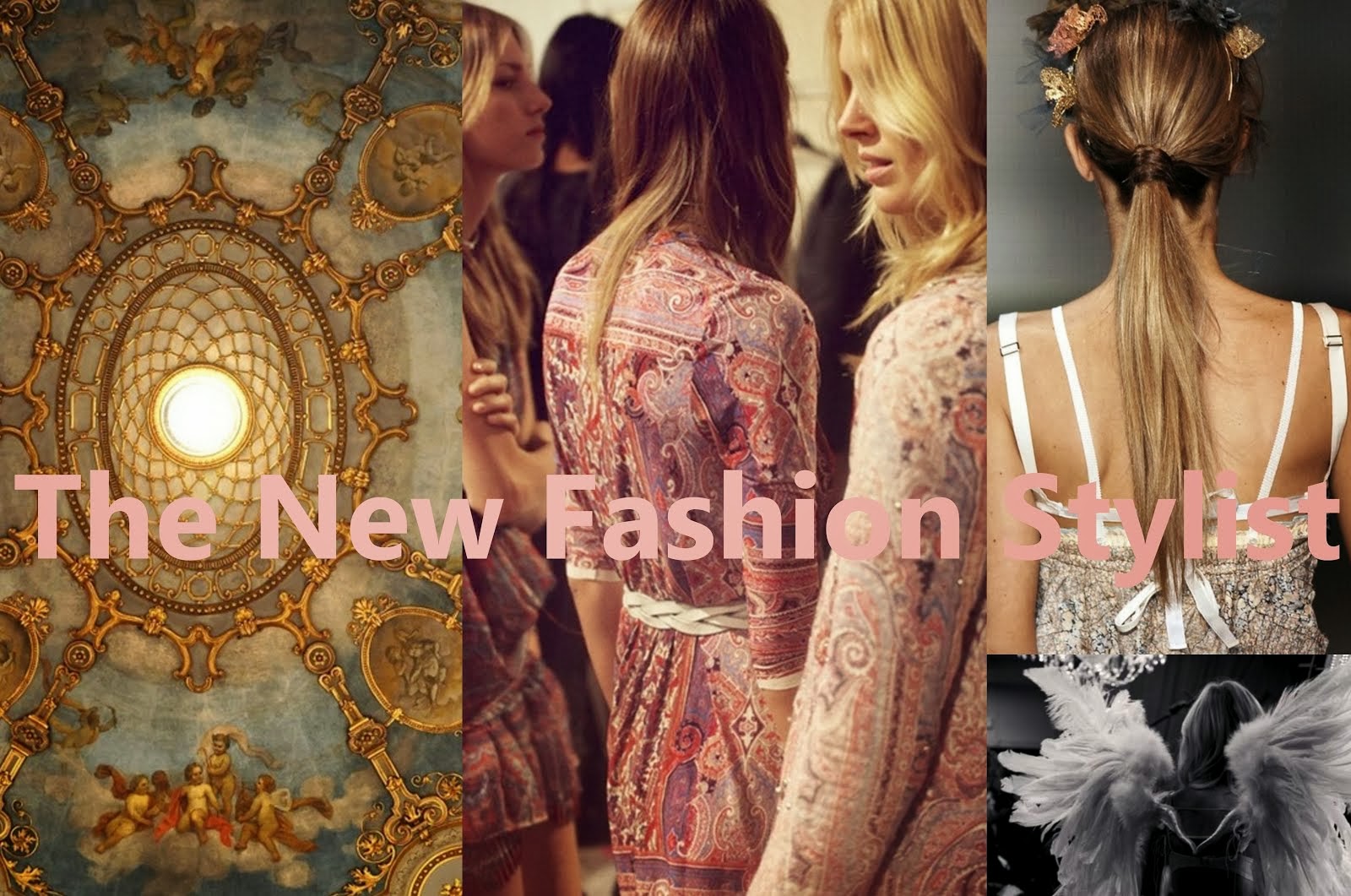A vibrant collage of three distinct sections, overlaid with large pink text reading "The New Fashion Stylist," spans the width of the image. On the left, a richly detailed section showcases a church ceiling adorned with intricate gold curlicues and frames, featuring paintings of baby cupids or cherubs nestled on a cloud against a blue backdrop. A prominent skylight in the center bathes the scene in light. The central section presents a fashion scene, with three young women in floral patterned dresses and long hair, possibly from a fashion show or magazine shoot. The right section highlights the back of a woman with her hair tied up, wearing a strapped dress that reveals much of her back; beneath her image is a black-and-white photograph of another woman, adorned with a striking pair of white angel wings. The collage is awash with colors including gray, black, pink, red, white, tan, purple, gold, and blue, enhancing the visual appeal of this fashion-centric montage.